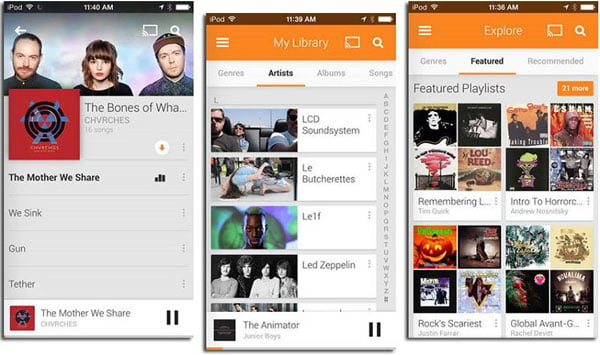These three screenshots provide an in-depth glimpse into an old iPod Touch app centered around music. At the top of each screenshot, the familiar “iPod” label resides in the top-left corner, accompanied by standard interface icons: a Wi-Fi symbol, a clock in the center, and a set of indicators on the right-hand side displaying location, Bluetooth connectivity, and battery life.

The first screenshot showcases the album "The Bones of What You Believe" by CHVRCHES. The album comprises 16 songs and features a header image of the band, highlighting the female lead vocalist alongside two male band members. The album cover stands out with its striking red background interlaced with three blue triangles and three interconnected black circles. The track "The Mother We Share" is currently playing, evidenced by three sound bars of varying heights. Beneath this, subsequent tracks are listed: "We Sink," "Gun," and "Tether." At the screen's bottom is the mini-player, reiterating that "The Mother We Share" by CHVRCHES is playing.

In the second screenshot, the music library is presented. Users are afforded the ability to sort their library by genres, artists, albums, or songs. The organization is alphabetical, as demonstrated by the scroll bar on the right displaying letters A to Z. The visible list includes bands like LCD Soundsystem, Le Butcherettes, Lykke Li, and Led Zeppelin, with "The Animator" by Junior Boys playing at the time of the screenshot.

The final screenshot delves into the explore page of the app. This section allows users to browse through various genres, featured playlists, and recommended playlists. Four sets of recommended playlists are visibly curated in this screenshot, suggesting a mix of musical exploration tailored to the user's preferences.

Overall, these screenshots not only illustrate the user interface of this nostalgic iPod Touch app but also capture the essence of discovering and enjoying music during its time.